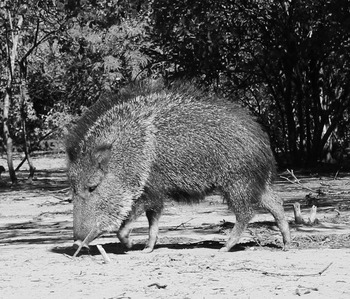This striking black and white photograph features a large warthog standing prominently at the center, occupying most of the frame. The warthog, facing towards the right side of the image, showcases its bristling fur, particularly along a dark mane that runs from between its small, laid-back ears down the ridge of its back. The foreground is a textured gray, possibly sand or dry grass, where the warthog appears to be rooting around with its snout, suggesting a search for food. Notably, its right eye is visible, adding a sense of alertness. The background is filled with dark, shadowy trees and some debris, emphasizing the wild and somewhat desolate environment. The animal’s shadow is cast distinctly, indicating a sunny day. The warthog's lean yet muscular build is evident in the definition around its shoulders and haunches, and there's no visible tail. Overall, the photo captures a moment of natural foraging behavior of this rugged and imposing creature.